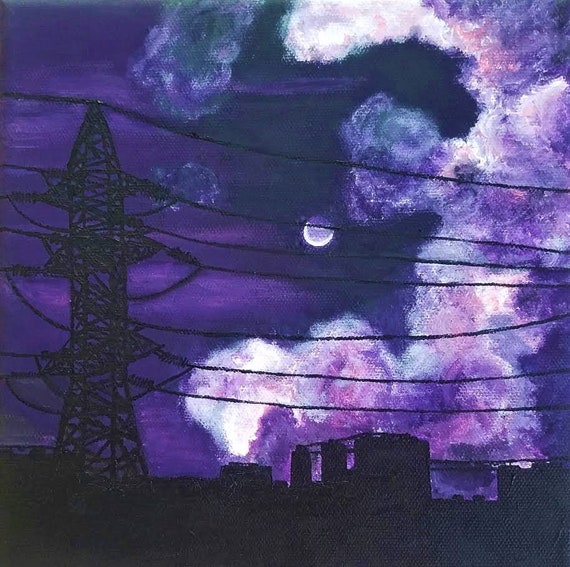This captivating watercolor painting portrays an evocative night scene dominated by high tension power lines stretching horizontally across the composition. At the center of the image, a full moon shines through a veil of purples, blues, and blacks, accentuating the mysterious atmosphere. A prominent electrical tower rises amidst the dark, shadowy sky, intersecting the moon with its cables. The background reveals an industrial factory, emitting white steam that curls up and around the right edge of the image, blending with the sky's varied purples and pinks.

Adding to the nocturnal ambiance, the sky is adorned with ominous clouds tinged with purples and whites, contributing to the overall dark and brooding aesthetic. In the distance, faint outlines of several buildings, including three tall structures, emerge through the dense shadows, reinforcing the industrial tone. Despite the intricate interplay of color and form, the details in the foreground and background remain deliberately obscure, enhancing the enigmatic quality of the scene.